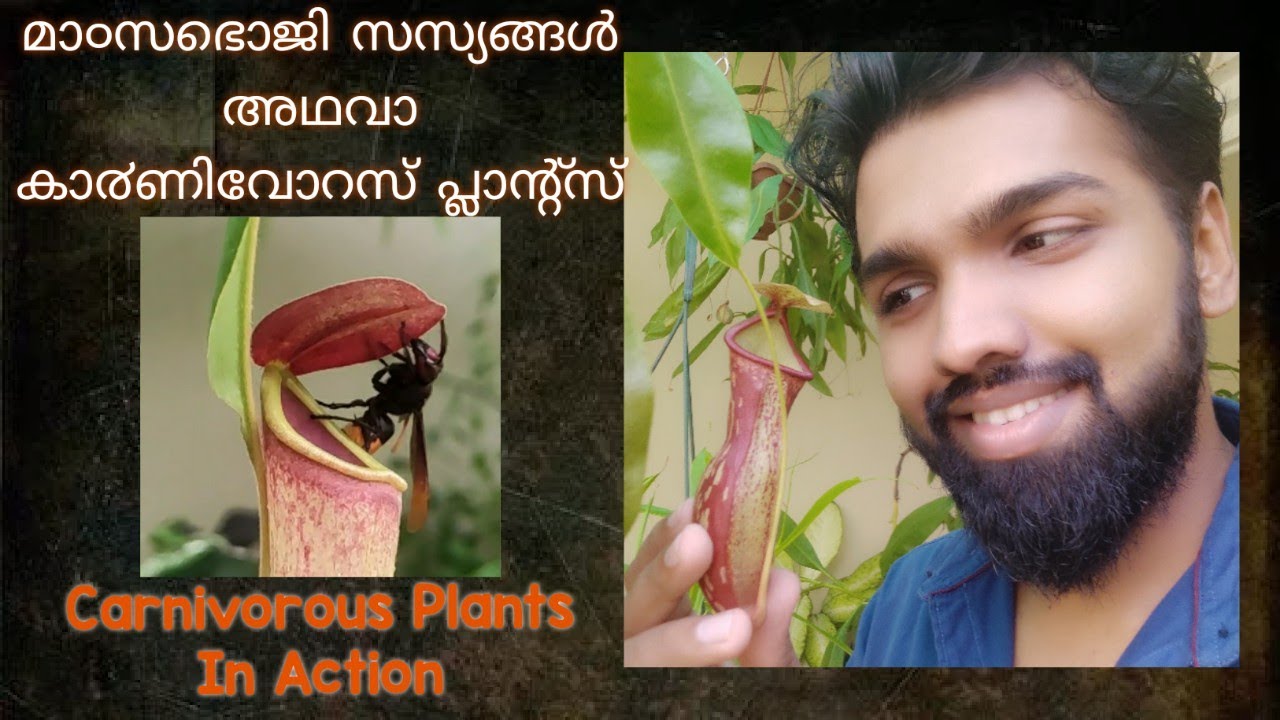The image features a collage on a black and gray background, showcasing an exploration of carnivorous plants in action. On the right, there is a photograph of a Middle Eastern or Indian man with tan brown skin, a black beard, and short, gelled black hair. He is wearing a blue collared shirt and smiling as he intently observes a plant he holds between his hands. This plant, which appears to be a Venus flytrap with red and light green hues, seems to be mid-action, possibly capturing an insect.

To the left, a smaller, square photograph offers a close-up view of the same plant. In this image, a wasp with black and copper-toned wings is seen approaching one of the plant's buds. Above this close-up, there is some white text in what seems to be Arabic script, providing additional context in a foreign language. Below the image, in orange text, the phrase "Carnivorous plants in action" can be seen, emphasizing the dynamic nature of the scene.